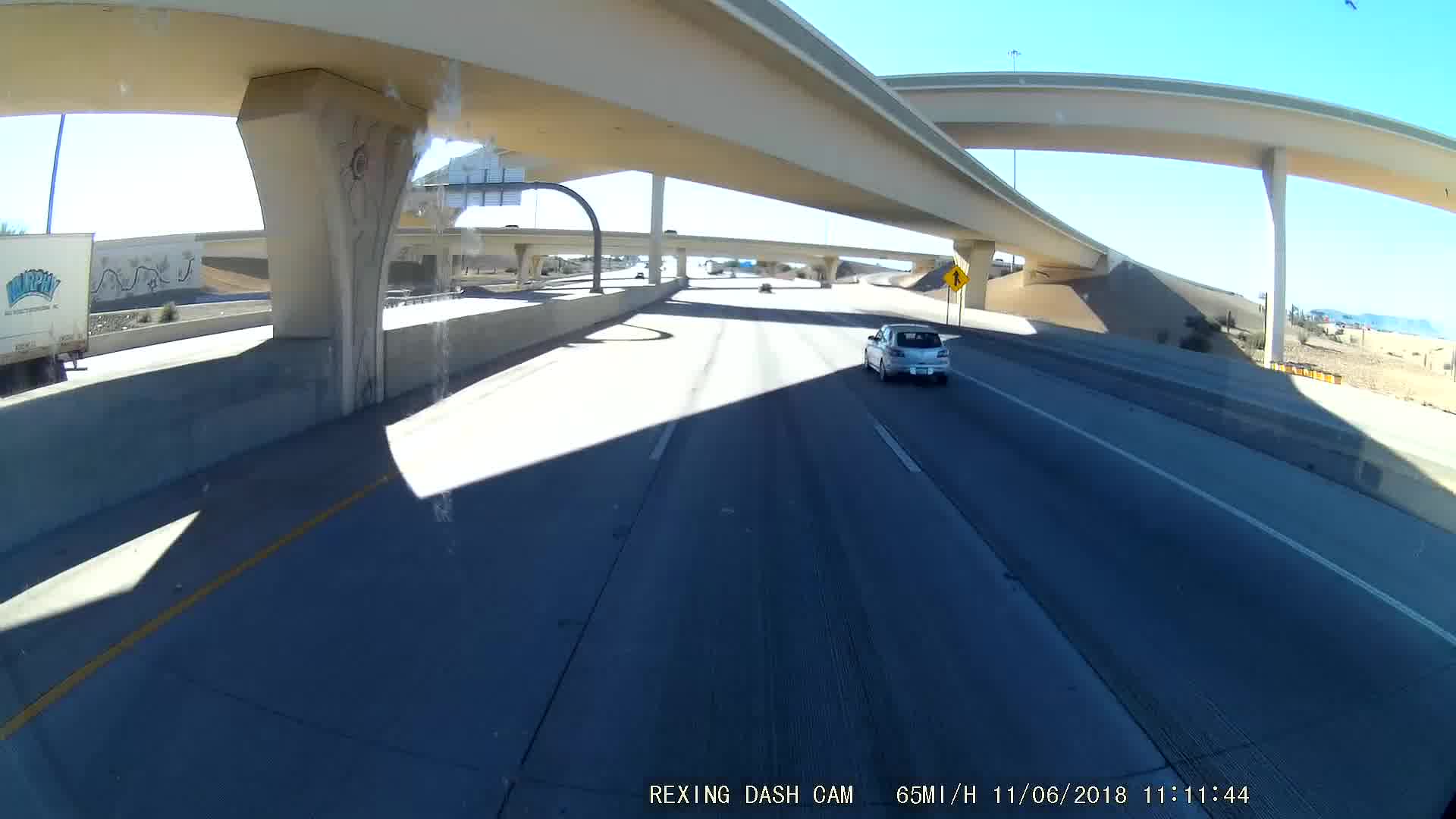The image is a photograph captured from a dashcam, taken on November 6, 2018, at 11:11:44 AM. It shows a three-lane freeway under a bright, sunny, teal blue sky with some clouds. The freeway features several overpasses: one directly overhead, another curving above at the top of the image, and two crossing each other about a quarter mile out. The scene includes a small silver car in the far right lane, covered in shadow, ahead of the dashcam vehicle which is presumably in the center lane. There is also a truck with a cube back, similar to but smaller than an 18-wheeler, visible on the left side of the freeway, driving in the opposite direction. The freeway is supported by dirt embankments and concrete pillars. The text at the bottom of the image reads "Rexing dash cam 65 mi/h" indicating the recording speed, along with the date and timestamp.